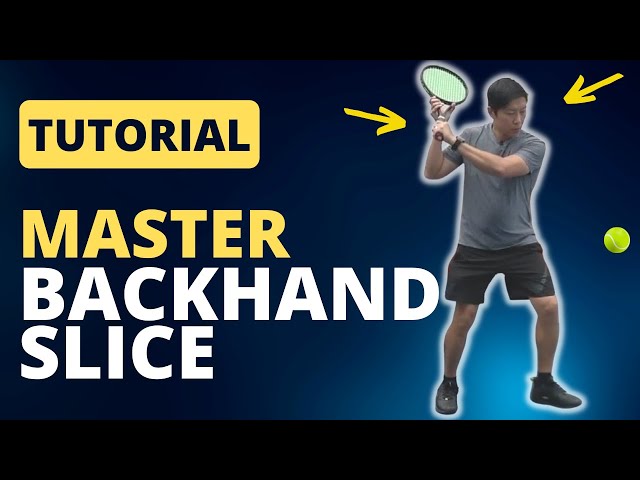The image depicts an Asian man ready to hit a tennis ball with a backhand slice. He is wearing black shoes, black socks, dark gray shorts, a short-sleeved gray t-shirt, and a watch with a black wristband. The man holds a tennis racket with both hands, pulling it back over one shoulder in preparation to hit a light green or yellow tennis ball hovering around his waist. The strings of the racket appear light green. Two yellow arrows point towards the man, one at his wrist and one at his head, highlighting key aspects of his form. The background is composed of different shades of blue, with a dark blue base hue. The text "Master Backhand Slice" is prominently displayed in large bold letters; "Tutorial" is positioned within a yellow rectangle in dark blue font, "Master" is in yellow, and "Backhand Slice" is rendered in white. The black horizontal stripe runs along the bottom edge of the image, contrasting with the overall blue tones. The detailed arrangement and setting suggest it is either a poster, book cover, or a thumbnail for a YouTube tutorial video.